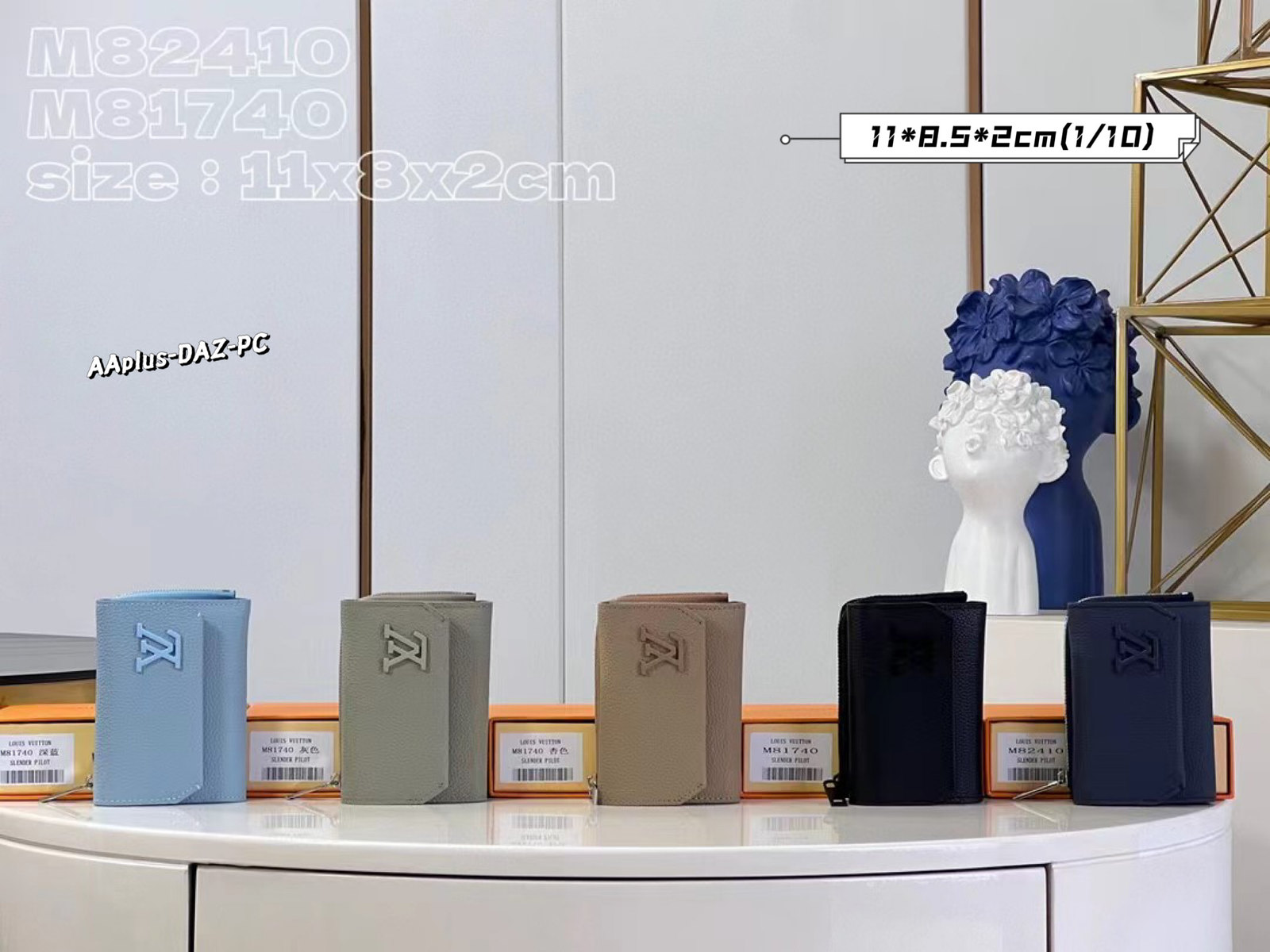This vibrant photograph features a pristine, minimalist setting, likely a display rather than a store. Front and center, we see a series of five Louis Vuitton wallets meticulously arranged atop a sleek, white porcelain countertop. Each wallet is paired with its respective box, featuring SKU labels and additional details. From left to right, the wallets are colored light blue, khaki, beige, black, and dark navy. The Louis Vuitton logo, in a distinct XL design, embellishes each wallet. The background boasts a stark white wall, accented by two thin, brown vertical lines. 

In the upper part of the image, to the far left, various labeled codes are displayed: M82410, M81740, and dimensions listed as 11x8x2 cm. Adding a touch of artistic flair, two stylized head statuettes with curly hair stand behind the wallets—one smaller and white, the other larger and dark blue. To the right of them, there are three see-through stacked cubes, connected by light brown frames, contributing an architectural element to the scene. Near this arrangement is a detailed label with the enigmatic inscription, "AAPLUS-DATZ-PC," alongside another rectangular bordered area housing additional numbers and codes. The meticulous setup, combined with clean lines and careful detailing, creates a sophisticated, almost gallery-like ambiance for this luxury brand display.